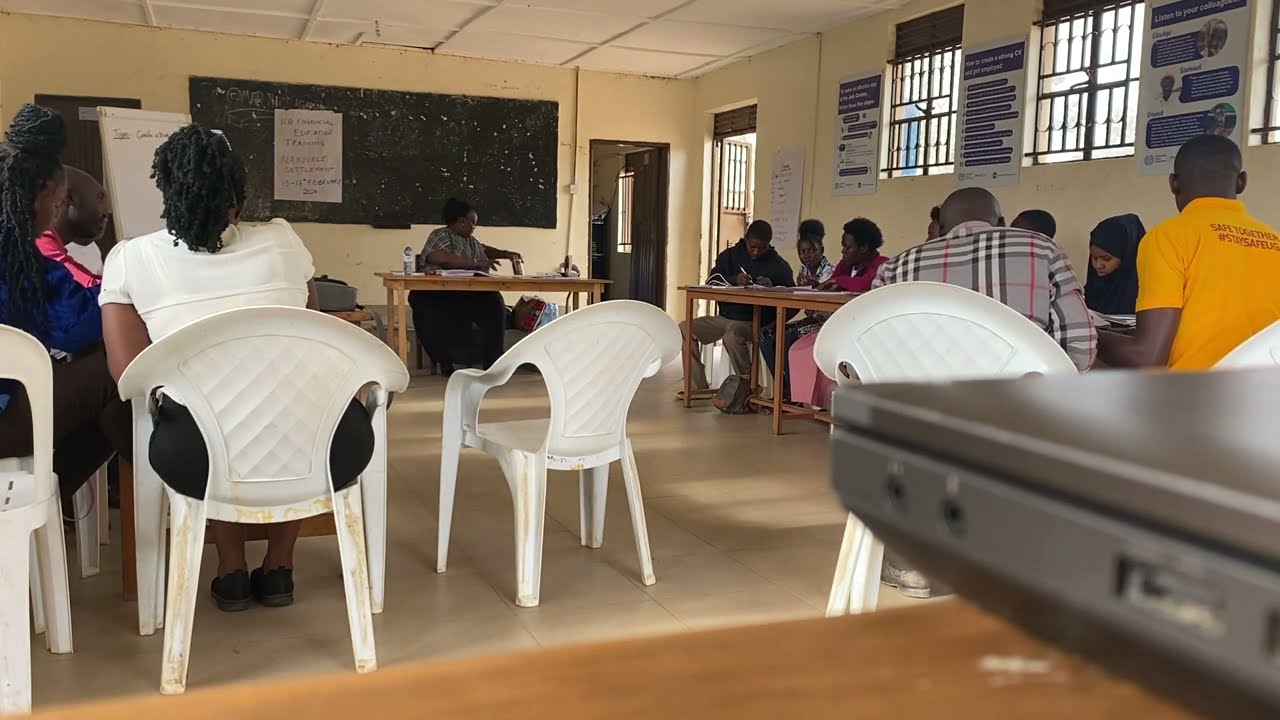The image captures a daytime indoor scene of what appears to be a classroom focused on career guidance. The room has light yellow walls with two barred windows on the upper right side, allowing sunlight to illuminate the space. In the right corner, an open door also lets light in, complementing the bright atmosphere. The classroom is arranged with a long wooden desk underneath the windows, where several people of African descent are seated, diligently writing on papers. These individuals are likely students, engaged in the learning material.

To the left side, more directly in front from the viewer’s perspective, a few women are seated on white plastic chairs with their backs to the camera. On the wooden table in front of these chairs, a closed silver laptop can be seen on the right side. The classroom features motivational posters, one of which encourages listening to colleagues, while another offers tips on creating a strong CV and gaining employment.

In the front of the room, a woman of African descent is seated at a wooden desk with a water bottle next to her. Behind her hangs a blackboard adorned with white papers containing English text, possibly related to financial education or career advice. Another door, which leads to an adjacent room, can be seen to the left of this desk. The blackboard and the posters reinforce the educational and career-oriented environment of the classroom.